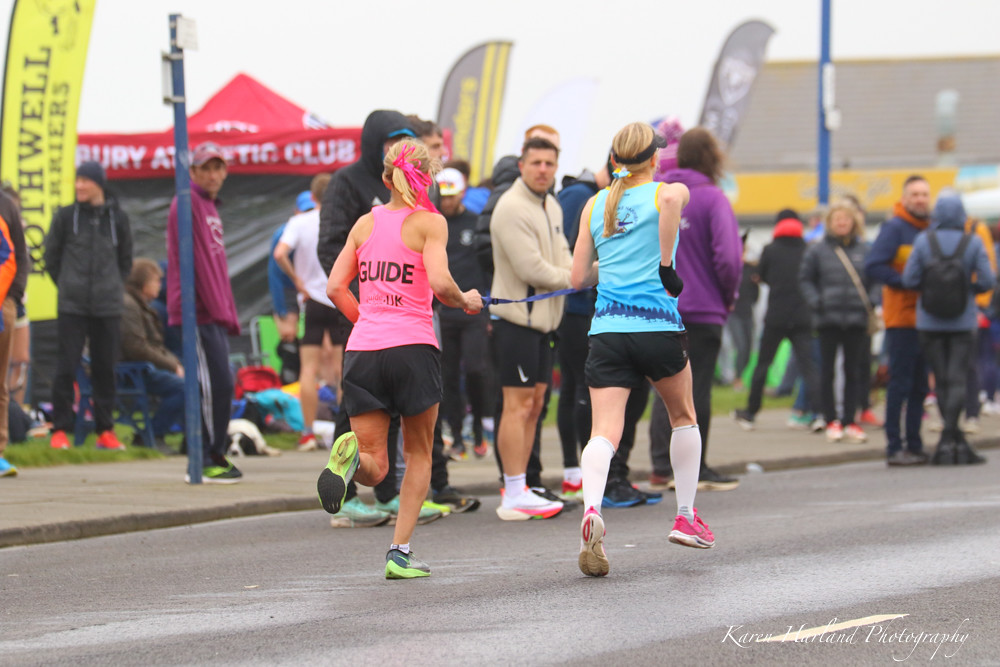In this vibrant outdoor photograph capturing the energy of a road race, two women with long blonde hair jog side by side, establishing a palpable sense of camaraderie through their synchronized strides. Both runners have their hair neatly tied back in ponytails, with the woman in the pink tank top distinguished by a long, hot pink ribbon and sporty green tennis shoes. The back of her tank top boldly displays the word "Guide." Her companion in a bright blue tank top, accentuated by a black visor, contrasts with knee-high white socks and pink tennis shoes. Clutched in the woman's hand is a blue lead, linking her subtly to the "Guide" in pink, underscoring the collaborative nature of their endeavor. Both wear black shorts as they navigate the road, surrounded by a bustling crowd. Spectators, warmly dressed in winter jackets, line the sidewalk, engaging in conversations, watching intently, and some carrying backpacks. Further back, a green grassy area dotted with tents and flanked by flags, including one yellow flag with the inscription "TH Well," brings added vibrancy to the backdrop, encapsulating the dynamic and lively atmosphere of the event.